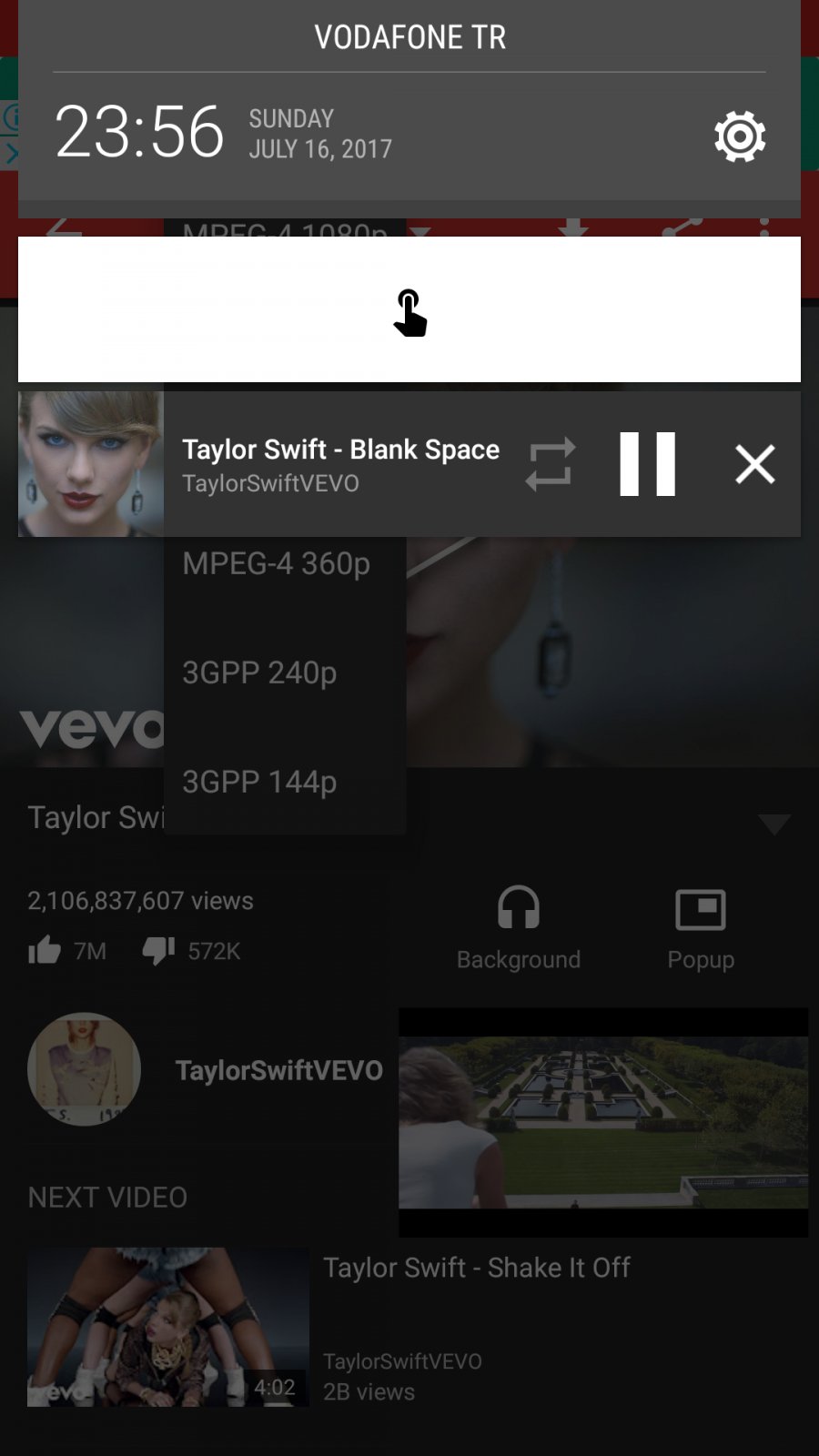This image depicts a tablet or smartphone screen full of notifications and user interface elements. At the top of the screen, a dark gray rectangle houses a series of elements: in the center, bold white text reads "ODEFRONTRBODAFONETR". On the left-hand side, the time is displayed in bold white text as "23:56," set to military time. Next to this, in gray text, are the details "SUNDAY, JULY 16, 2017" in all caps. On the right-hand side, there is a bold white gear icon indicating settings.

Below this, a white rectangle features a black fingertip icon within a black circle, indicating a touch interaction. Underneath, there is a media player interface within a dark gray rectangle. On the left, an image of Taylor Swift is shown wearing emerald earrings, with her name and song title "Taylor Swift - BLACKSPACE" in bold white text. Below this, in gray, it says "Taylor Swift VEVO".

To the right of the song details, there are shuffle controls: an arrow pointing right with a descending line and an arrow pointing left with an ascending line. Additionally, two bold white lines symbolize the pause function, and a white "X" indicates an option to exit the song. Below the media controls is a black band displaying available video quality options: "MPEG-4 360p, 3GPP 240p, and 3GPP 144p."

The background prominently features "VEVO" in bold white text and "Taylor Swift" underneath it. The video has amassed 2,106,837,607 views, 7,000,000 likes, and 572,000 dislikes. An icon of headphones in bold white text accompanies the word "BACKGROUND" in gray, and next to it is a double-square icon labeled "POP UP" in gray. The screen also shows an image of Taylor Swift, with the top of her head slightly cropped, and the label "Taylor Swift VEVO."